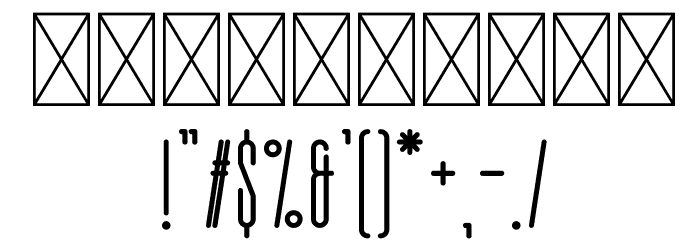The image features a series of ten elongated black boxes arranged in a horizontal layout. Each box has a prominent white outline and contains a large white 'X' traversing from the top corners to the bottom corners, intersecting in the middle. Below these boxes is a row of various bolded punctuation characters. The characters appear elongated and each has a distinctive style. From left to right, the characters include:

1. Exclamation mark (!)
2. Double quotation marks (")
3. Pound symbol (£)
4. Number sign (#)
5. Percentage sign (%)
6. At sign (@)
7. Ampersand (&)
8. Single apostrophe (')
9. Parentheses (())
10. Asterisk (*)
11. Plus sign (+)
12. Comma (,)
13. Minus sign (-)
14. Period (.)
15. Backslash (\)

Each character is displayed clearly, contributing to an organized and visually striking lower section of the image.